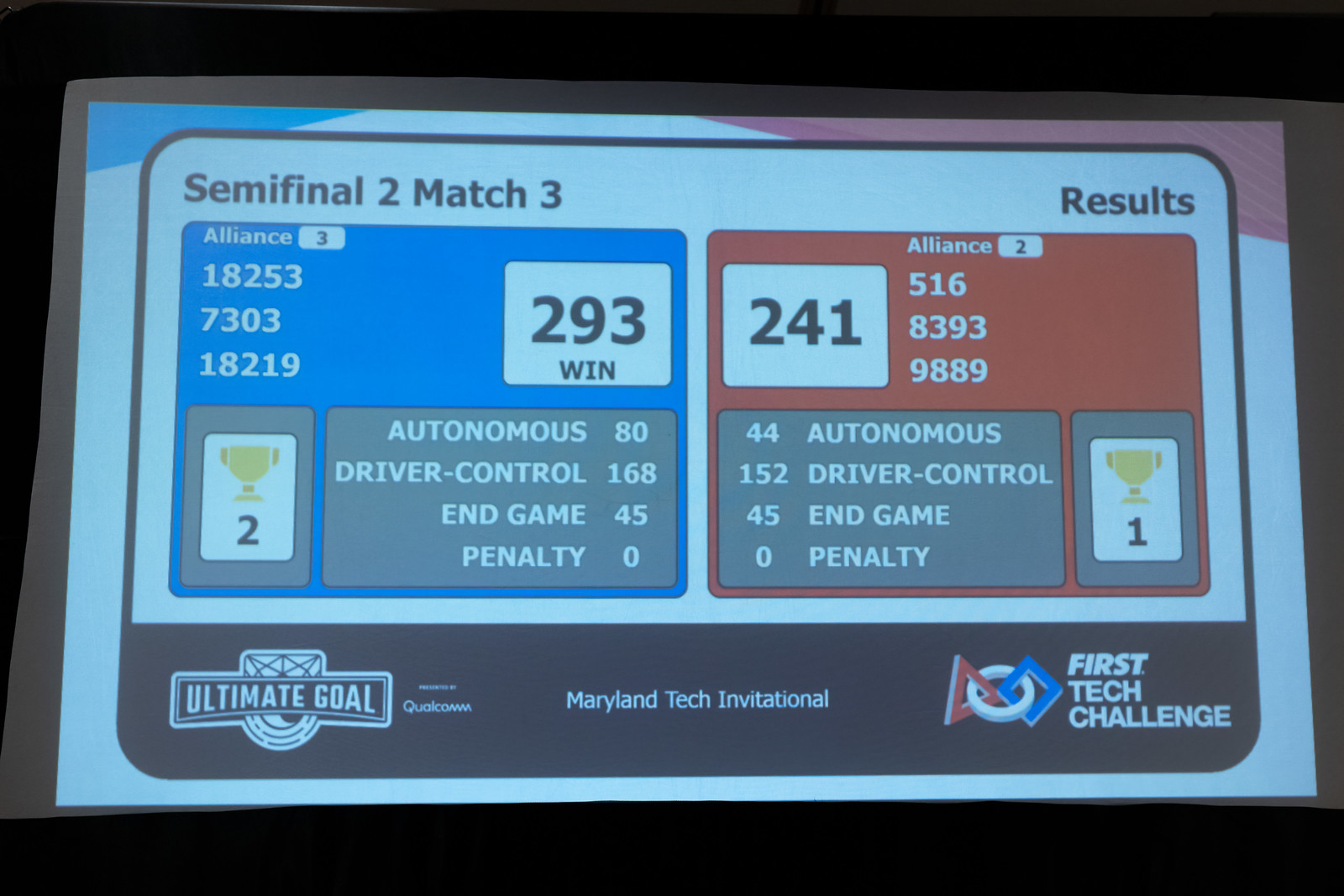The image depicts a digital screen showing the results of Semifinal 2, Match 3. The screen is divided into two sections: a blue-background rectangle on the left and a red-background rectangle on the right. The blue section represents Alliance 3, with a total score of 293 points broken down into 80 points for autonomous, 168 for driver control, and 45 for endgame, with no penalties. Additionally, it shows two trophies. The red section represents Alliance 2, with a total score of 241 points, consisting of 44 for autonomous, 152 for driver control, and 45 for endgame, also with no penalties, and one trophy. At the bottom of the screen, beneath these sections, is a banner featuring text that reads "Ultimate Goal" over a top-down illustration of a goal net. Central to the banner is "Maryland Tech Invitational," and the bottom right corner has the "First Tech Challenge" logo. The entire display is surrounded by a thin black border.